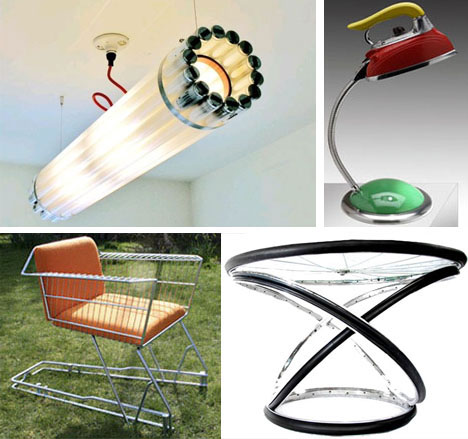This is a photograph depicting four unique, potentially handmade pieces of furniture or decorative items. In the upper left corner, a tubular light fixture composed of smaller white tubes is held together with metal bands and hangs by red and black extension cords from a white ceiling. The room is entirely white, giving a stark contrast to the light fixture. Adjacent to it on the right, a quirky desk lamp features a red iron with a yellow handle attached to a curved silver bar that extends from a green base. In the bottom left-hand corner, an artistic chair is crafted from a shopping cart with orange cushions placed inside the cut-off cart to form a comfortable seat. To the right of that, a modern table with a clear glass, pizza slice-shaped top is supported by an intricate base of swirling black legs that wrap around it, creating a striking hourglass-like form.